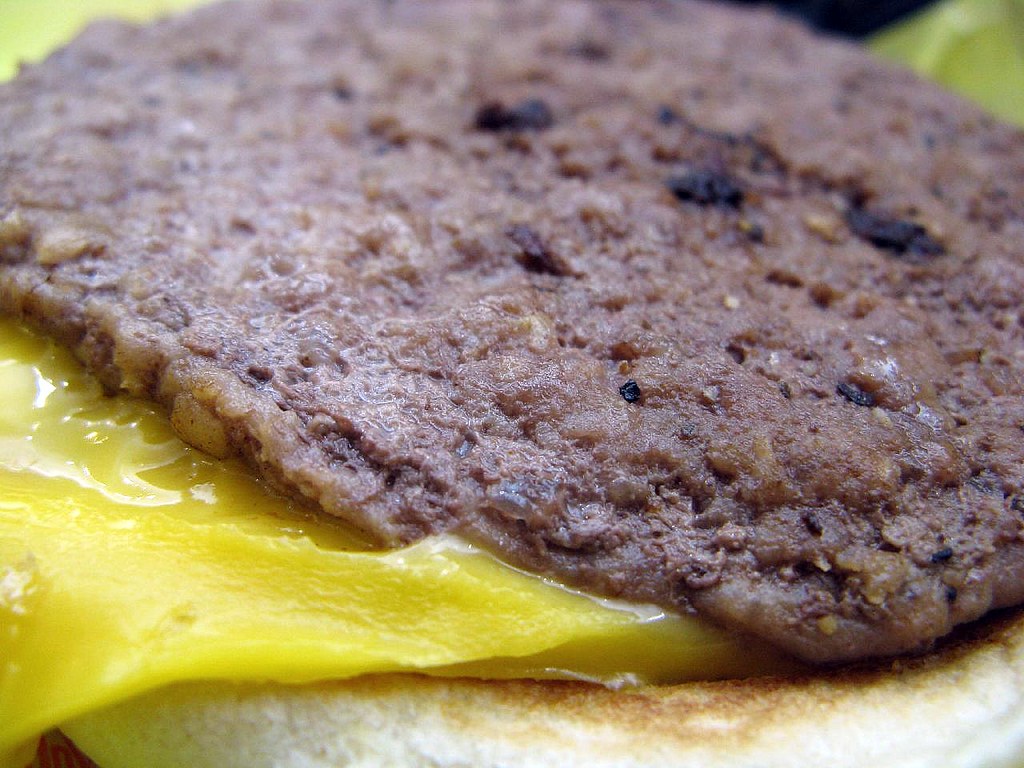This extremely close-up photograph showcases a well-done hamburger patty prominently positioned at the top of the image. The patty itself is largely brown with scattered spots of black, yellow, and brown throughout. Beneath the patty, a layer of cheese appears bright yellow and gooey, some parts melty and some harder, likely having started to cool around the edges. The cheese rests on what looks like an English muffin, displaying a predominantly white surface with some browning indicative of griddle marks. Only the cheeseburger dominates the frame, though a small, out-of-focus yellow section appears in the top right corner, potentially suggesting yellow paper commonly found in food baskets. The background beyond the main subject is largely black, providing a stark contrast and ensuring the patty remains the primary focus.